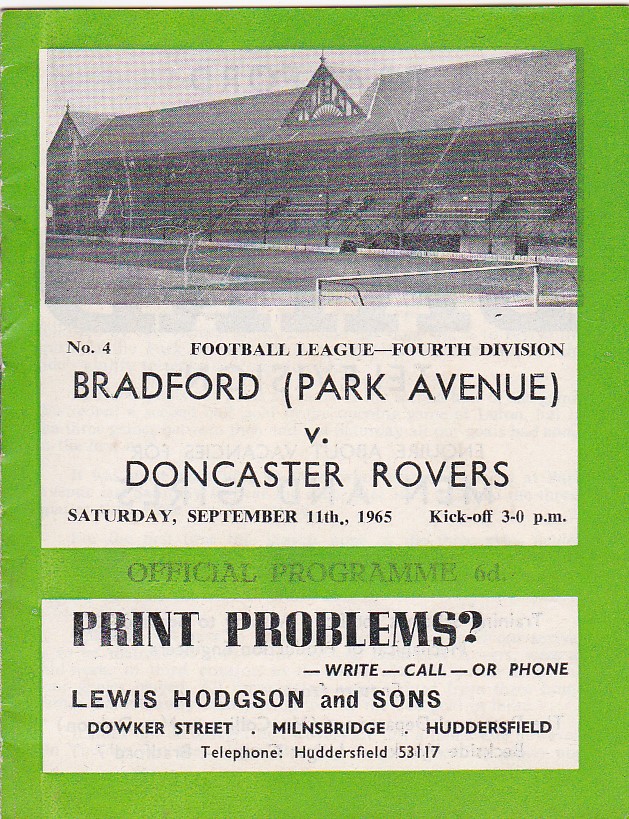This black and white front page of a football league program is set against a striking lime green background. At the top of the page, there is a vintage black and white image of an outdoor football arena. This image prominently features the stadium stands, which are partially covered by a roof, with a few scattered spectators visible. Below it, the fenced football field is displayed, along with one of the goals positioned on the right-hand side.

Central to the page, in bold black text set against a white background, the program details read: "Number Four Football League - 4th Division, Bradford Park Avenue vs. Doncaster Rovers, Saturday, September 11th, 1965, Kickoff 3 p.m., Official Program 6D."

At the bottom, an advertisement printed in black on a white background addresses printing needs and reads: "Print problems? Write, call, or phone Lewis Hodgson and Sons, Dowker Street, Milnes Bridge, Huddersfield. Telephone: Huddersfield 53117."